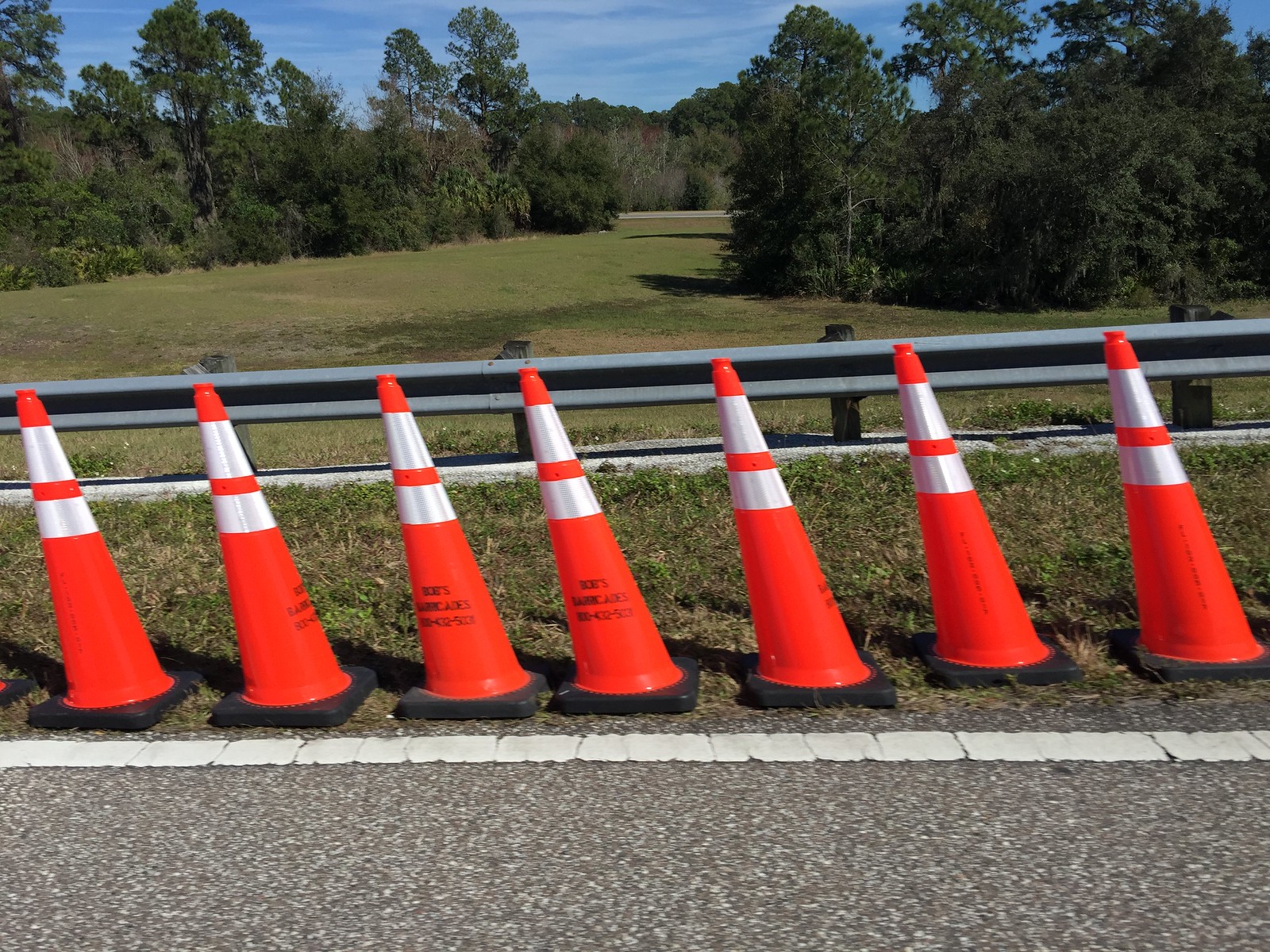In this image, a series of seven traffic cones line the side of a road. At the bottom of the image, a gray road is bordered by a solid white line marking its outer edge. Immediately behind the line, the traffic cones are upright, each featuring a black square base. The cones display a typical design of alternating colors: orange at the bottom, a white stripe, then orange again, another white stripe, and capped with orange tips. Behind the cones stretches a strip of green grass extending horizontally across the scene. Further back stands a gray railing, with an expansive grassy field beyond, receding into the distance. The landscape is framed by green trees on both sides, under a clear blue sky.